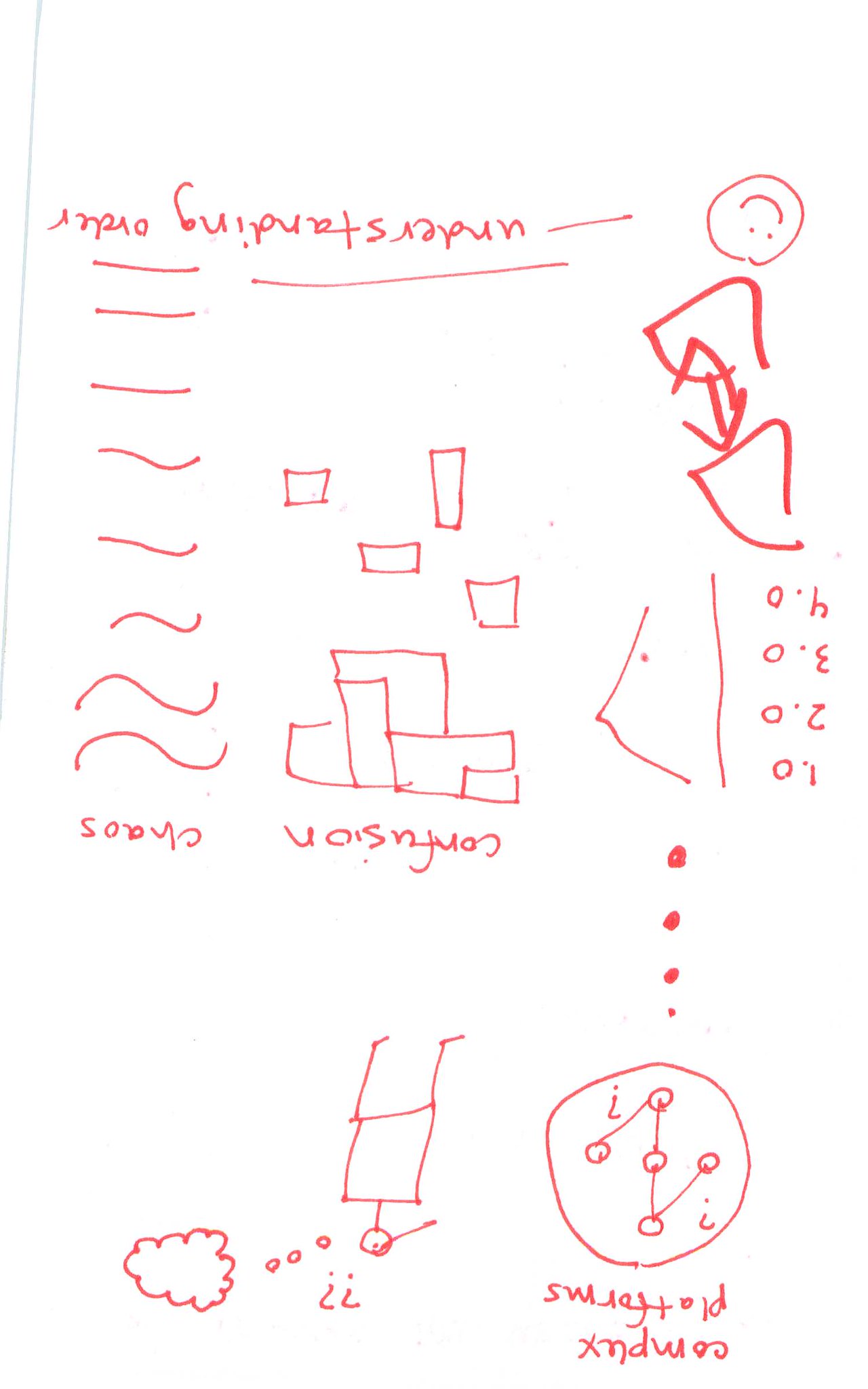The image is a detailed sketch featuring various diagrams outlined in red, all set against a white background. In the bottom left corner, there is a cloud-like shape highlighted in red. Surrounding this shape are three small red dots and a couple of upside-down question marks.

Adjacent to these elements, there's a unique structure consisting of a circular object, a vertical line, a square, and an open square stacked on top of each other. Moving to the right, a circle with five interconnected dots is depicted, accompanied by red upside-down text beneath it.

The diagram also includes four additional red dots, a sideways L shape, and a vertical line. There is a sequence labelled "1.0, 2.0, 3.0, 4.0," an arrangement of two triangles with arrows pointing between them, and an upside-down smiley face encircled by a circular shape.

To the left side of the diagram, a series of rectangles are arranged to form a singular figure. Adjacent to this, another word is noted, followed by a pattern of eight curvy, wavy lines that turn horizontal at their top ends. Above these lines, more red upside-down text is present, accompanied by a singular horizontal line below it.